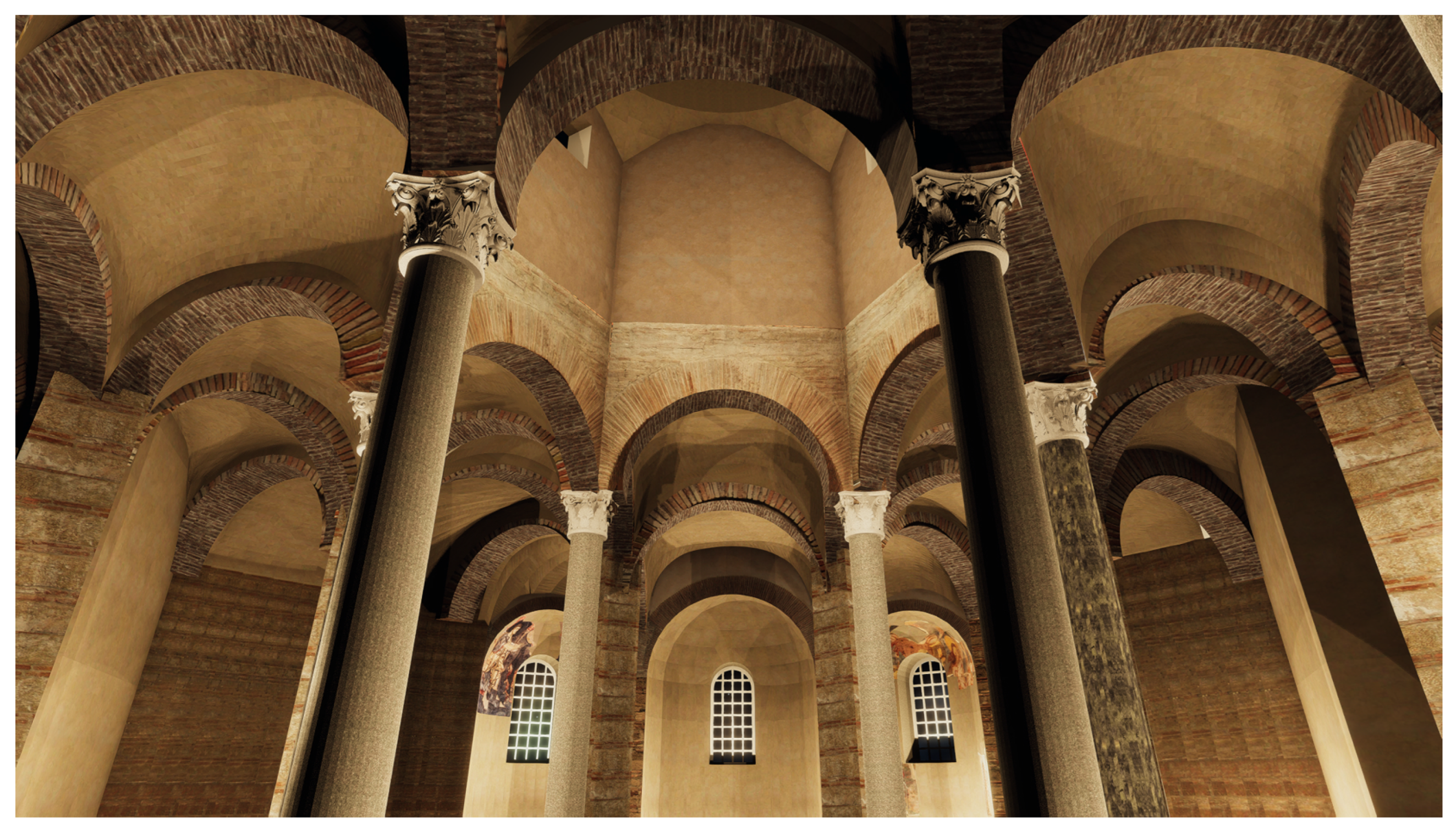The image captures a grand, well-preserved architectural interior that appears to be part of an ancient or historic building, characterized by its warm, earthy tones of beige, brown, and golden hues. The photograph, taken from ground level at an angle looking upward, showcases a series of towering Grecian-style columns. These columns, made of materials that resemble brick and possibly marble, support an intricate, arched dome ceiling adorned with complex awnings and archways.

In the foreground, two large, sculpted columns dominate the view, but it becomes evident that there is a circular arrangement of perhaps six columns extending beyond that. This arrangement creates a rhythmic pattern of arches connecting each column. Above, the ceiling features a light brown dome, further embellished with decorative elements.

Towards the lower part of the photograph, three long, rectangular windows with curved tops draw attention; they are framed by what might be murals or paintings around the windows on the left and right. The central window, however, is devoid of such decorations, displaying a clean, white picket paned effect that contrasts with the muted tones of the building.

The entire scene is bathed in ample light, highlighting the immaculate preservation and the detailed craftsmanship of this opulent architectural wonder.